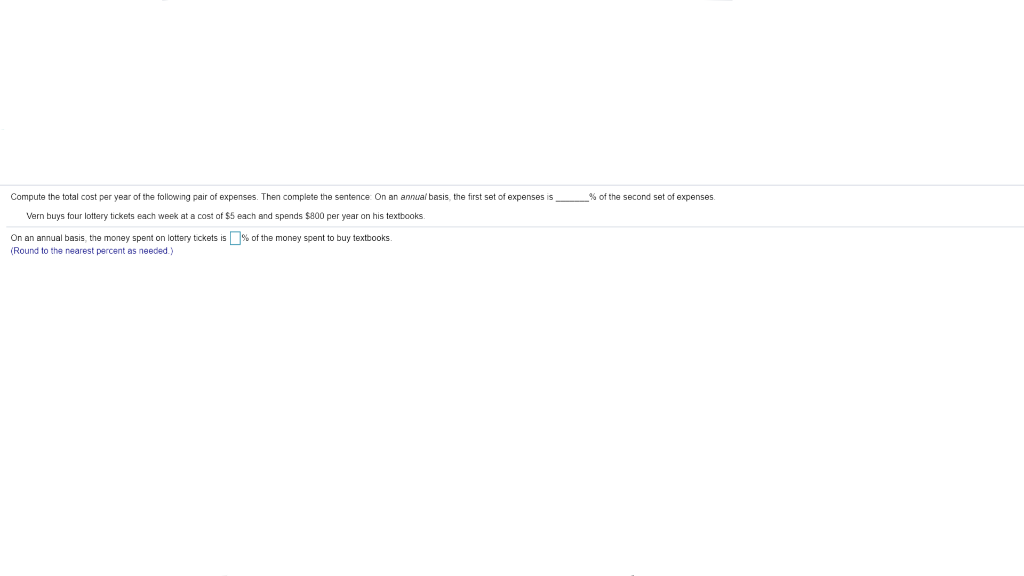The image is set against a white background and features a rectangular box with a white interior. The box's borders are gray, though only the top and bottom borders are visible as the left and right sides are cut off. Inside the box, in black text, it reads:

"Compute the total cost premiums of the following pair of expenses. Then, complete the sentence: On an annual basis, the first set of expenses is ______ percent of the second set of expenses."

Below this, the text continues:

"Vern buys four lottery tickets each week at a cost of $5 each. He spends $800 per year on his textbooks."

A gray line extends horizontally across the box, and beneath this line, the text reads:

"On an annual basis, the money spent on lottery tickets is ______ percent of the money spent to buy books."

At the bottom of the box, in blue text, it states:

"Round to the nearest percent as needed."